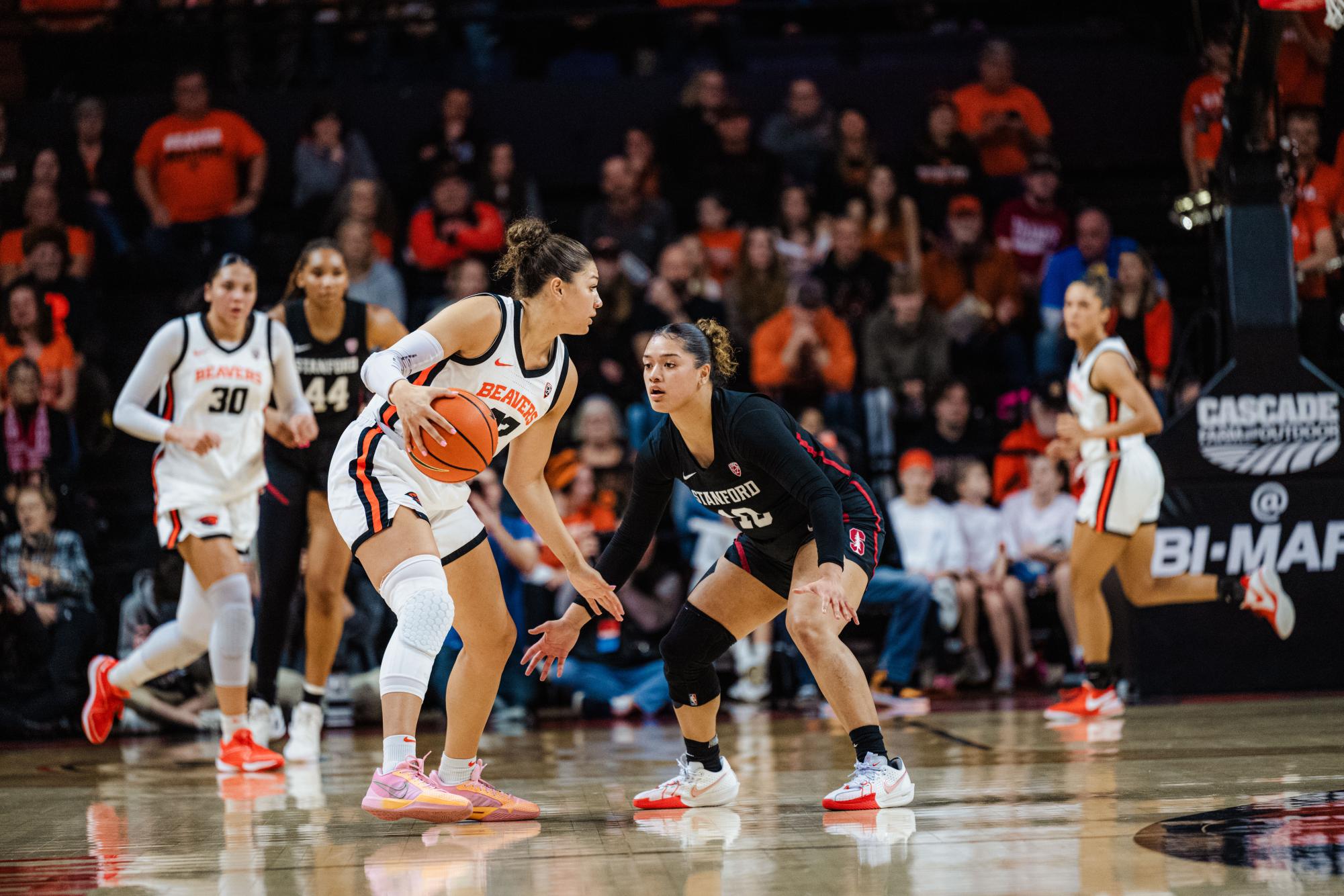This detailed action shot captures an intense moment in a women's college basketball game between Stanford and the Beavers. At the center of the image, a Beavers player, identifiable by her white uniform with orange and black stripes, is poised to dribble or pass the ball. She sports a knee brace on her right knee and striking pink sneakers. Facing her is a determined Stanford defender in a long-sleeve black uniform with red accents, attempting to block the play. The photo beautifully captures the dynamic energy of the game, with other players from both teams visible mid-run in the background. The glossy, pine-colored court is prominently seen at the bottom. In the blurred background, spectators fill the tiered seating, most clad in orange, presumably to support the Beavers. The basket is positioned in the back right, though the hoop itself isn't clearly visible. The scene conveys a palpable sense of anticipation and excitement, emblematic of a thrilling basketball match.